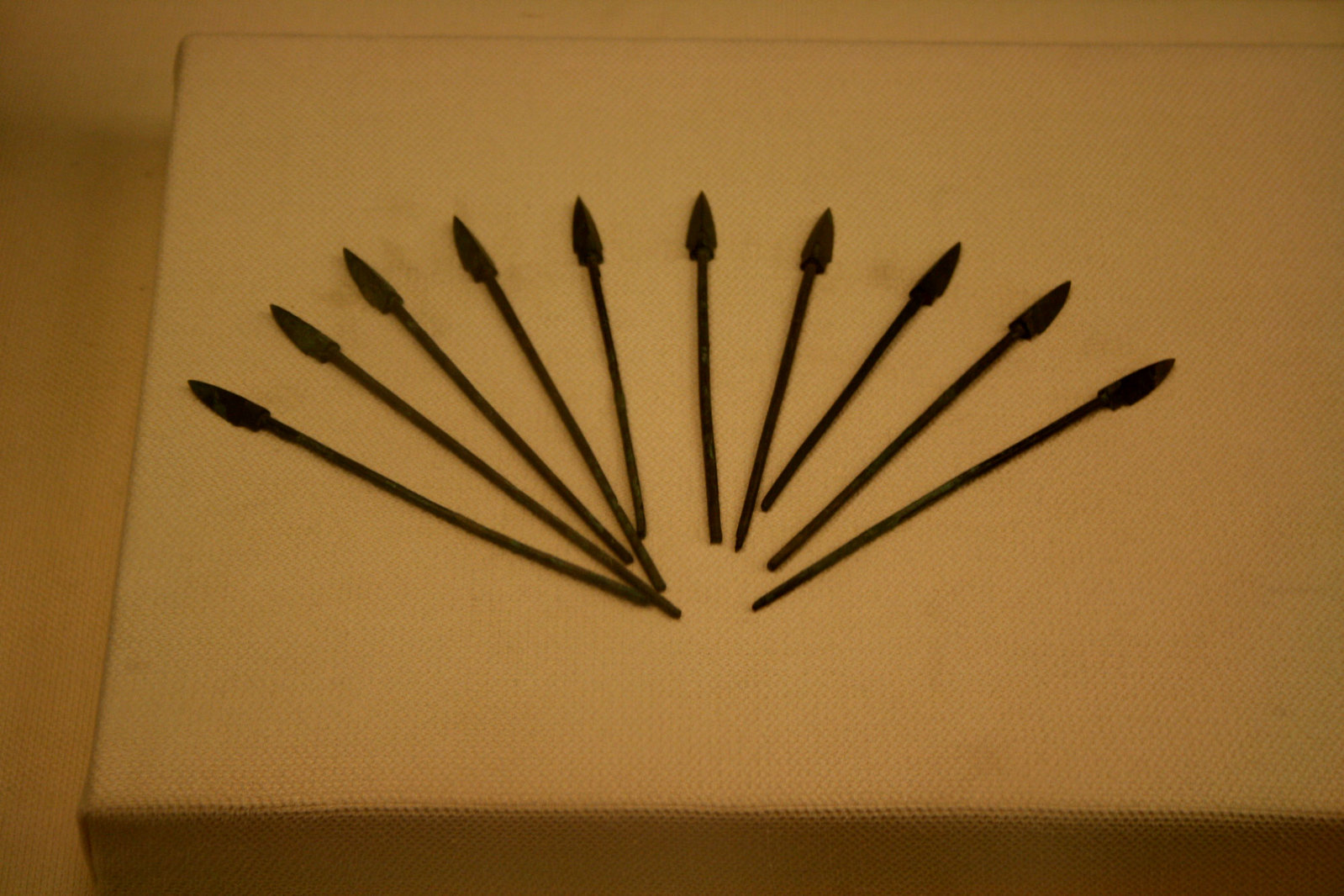This image captures ten primitive, dark brown or black objects resembling small spears or Native American arrowhead points with thin metal-like stems. They are meticulously arranged in a fan-like formation, nearly forming a half-circle. The points are displayed on a textured, white painting paper positioned on a tan or light brown surface that appears to be fabric. The display is more towards the left side of the paper, leaving some empty space visible on the left and top edges. The two objects on either end are positioned lower, while the two in the middle point straight up, creating a swooping effect. There's slight variation in the sizes, with some handles touching each other towards the left-hand side, while those on the right are spaced out but close. The image also hints at a blurred tan or light brown floor beneath the display surface, adding depth to the scene. Faint shadows cast by the spear-like objects enhance the detail and texture of the overall arrangement.